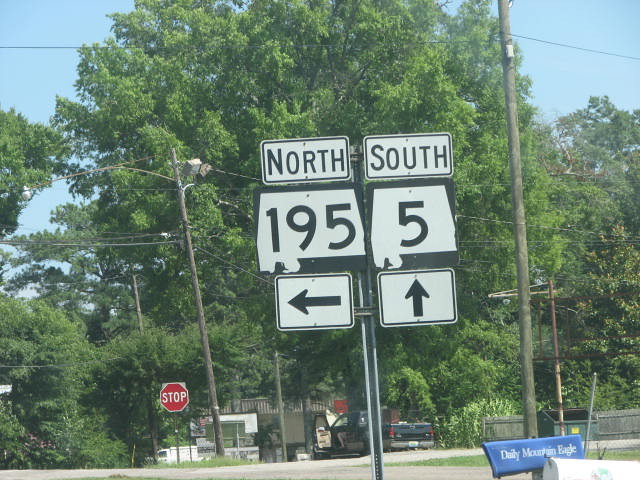This is a detailed digital color photo taken outdoors in a small town or neighborhood, showcasing a variety of elements under a clear, baby blue sky. The scene is dominated by lush trees, likely maple or oak, that fill the background with vibrant greenery. Prominently featured in the center of the image is a metal pole adorned with various street signs. The top-left sign is a white rectangle with a black border reading "North," and below it, a black square with the number "195" and the shape of a state, accompanied by a black arrow pointing left. On the right, a matching set indicates "South 5" with a black arrow pointing straight up. To the far left, a red octagonal stop sign is visible. In the foreground, towards the bottom right of the image, there is a white mailbox labeled "Daily Mountain Eagle" in gold font. Adjacent to it is a black paper box with the same inscription. The setting includes additional elements such as power lines, streetlights, and an empty bench, contributing to the suburban landscape. No people are present in the photo.